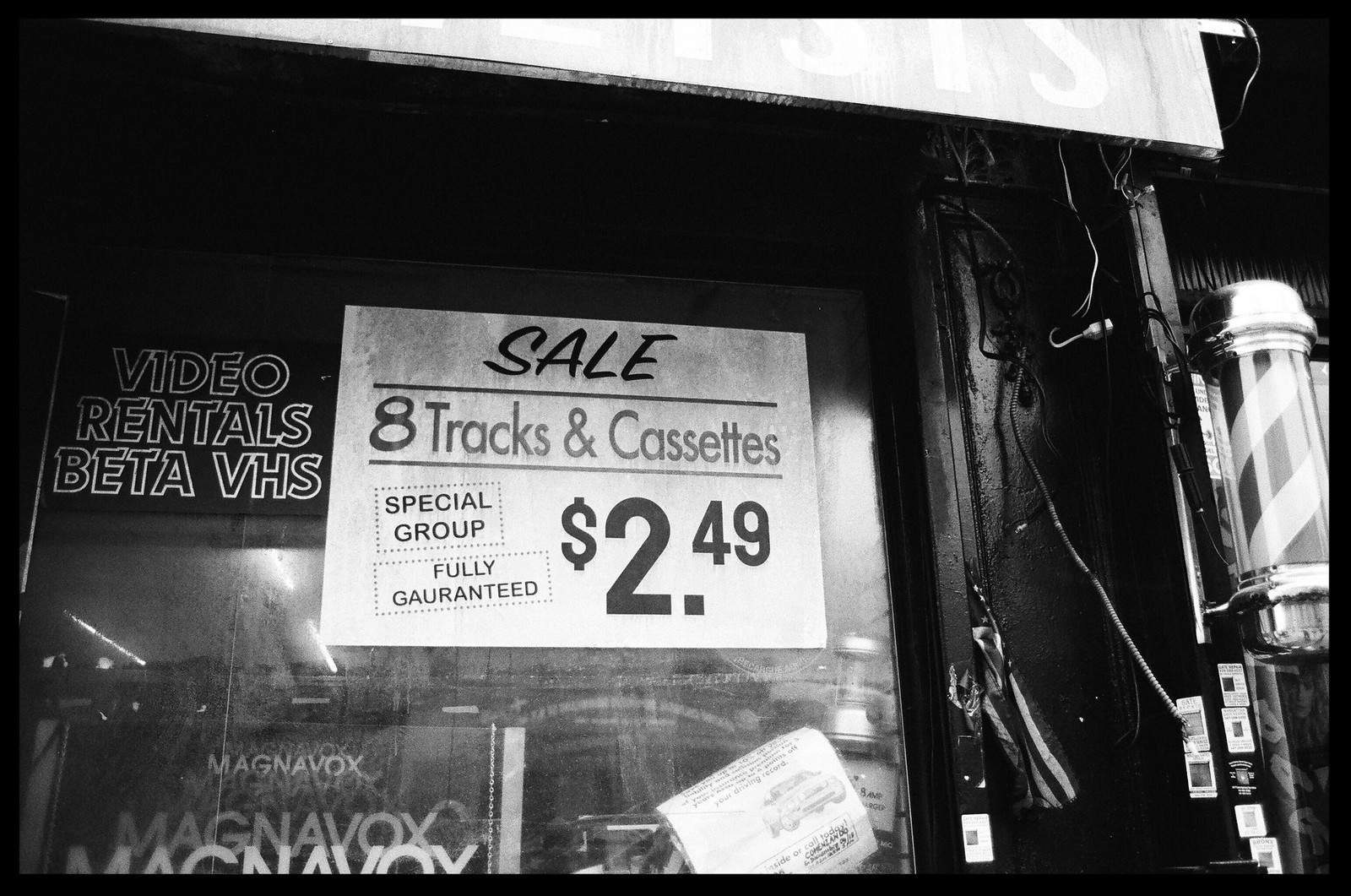This black-and-white image, framed with a thin black border, depicts the exterior window of a barbershop taken at night. Dominating the right-hand side is the iconic black-and-white striped barber pole. Several signs are affixed to the cloudy window: at the top left corner, a decal reads "Video Rentals Beta VHS"; beneath this, a smaller sign says "Magnavox." Centrally placed, a prominent white sign announces a "Sale" of "Eight Tracks and Cassettes," detailing "Special group, fully guaranteed, $2.49" in bold black letters enclosed in dotted black squares. The photograph's moody nighttime setting enhances the overall contrast, making the text and elements on the window stand out against the obscured interior.